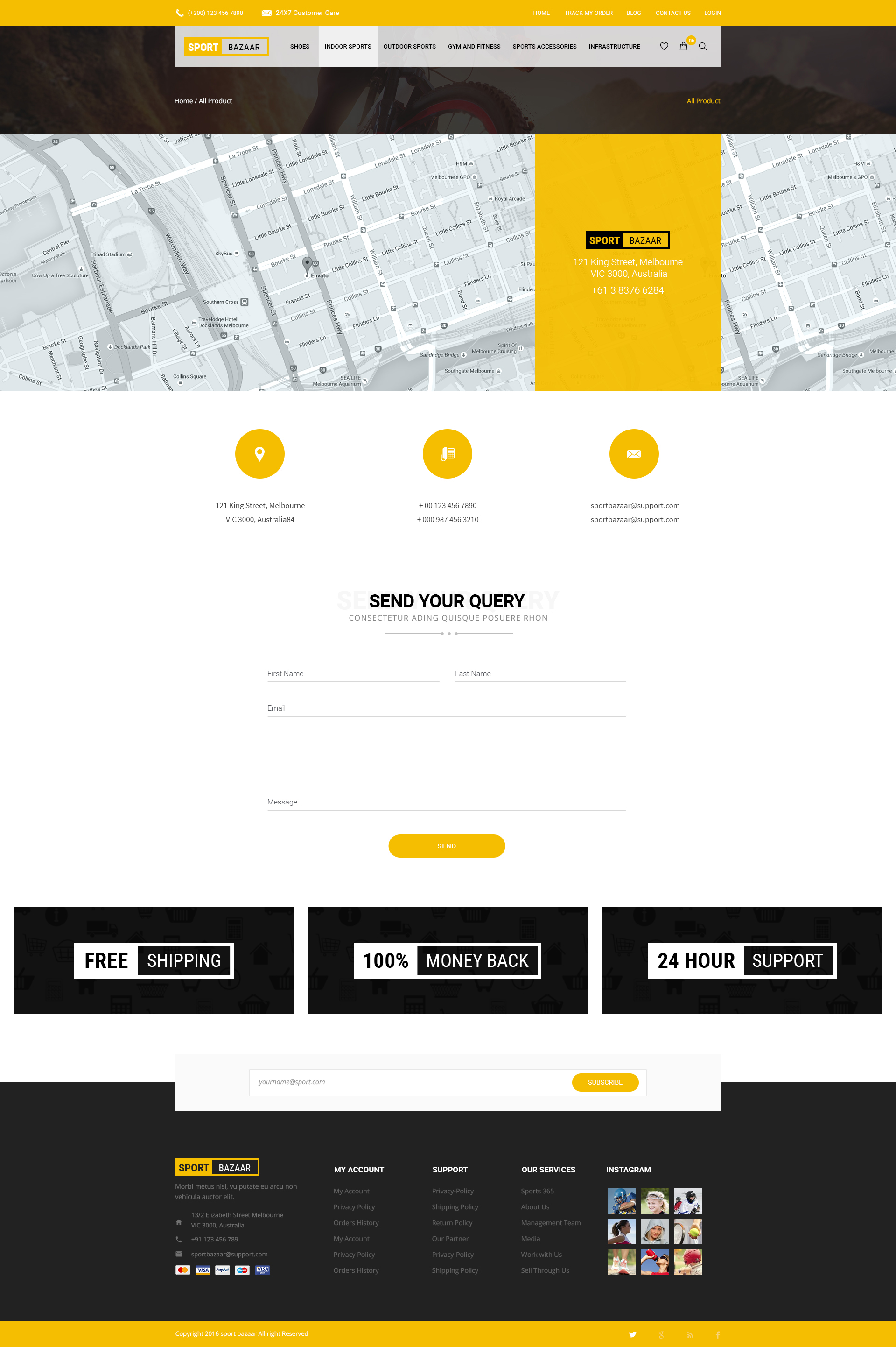This image captures the webpage layout of a sports bazaar website. Centrally at the top, there's a prominent menu bar showcasing the title "Sport Bazaar." Above this menu, a yellow horizontal bar stretches across the image, displaying a phone number in white text, possibly with additional menu items, although the text appears small. The central gray menu bar features six horizontally arranged menu options. At the far right end of this bar, there are three icons: a heart representing favorites, a shopping cart for purchases, and a magnifying glass for search functionality. Below the menu bar, there's an aerial view of a map with a GPS marker indicating a specific address. Beneath the map, three yellow buttons are visible, likely for navigation or action purposes.